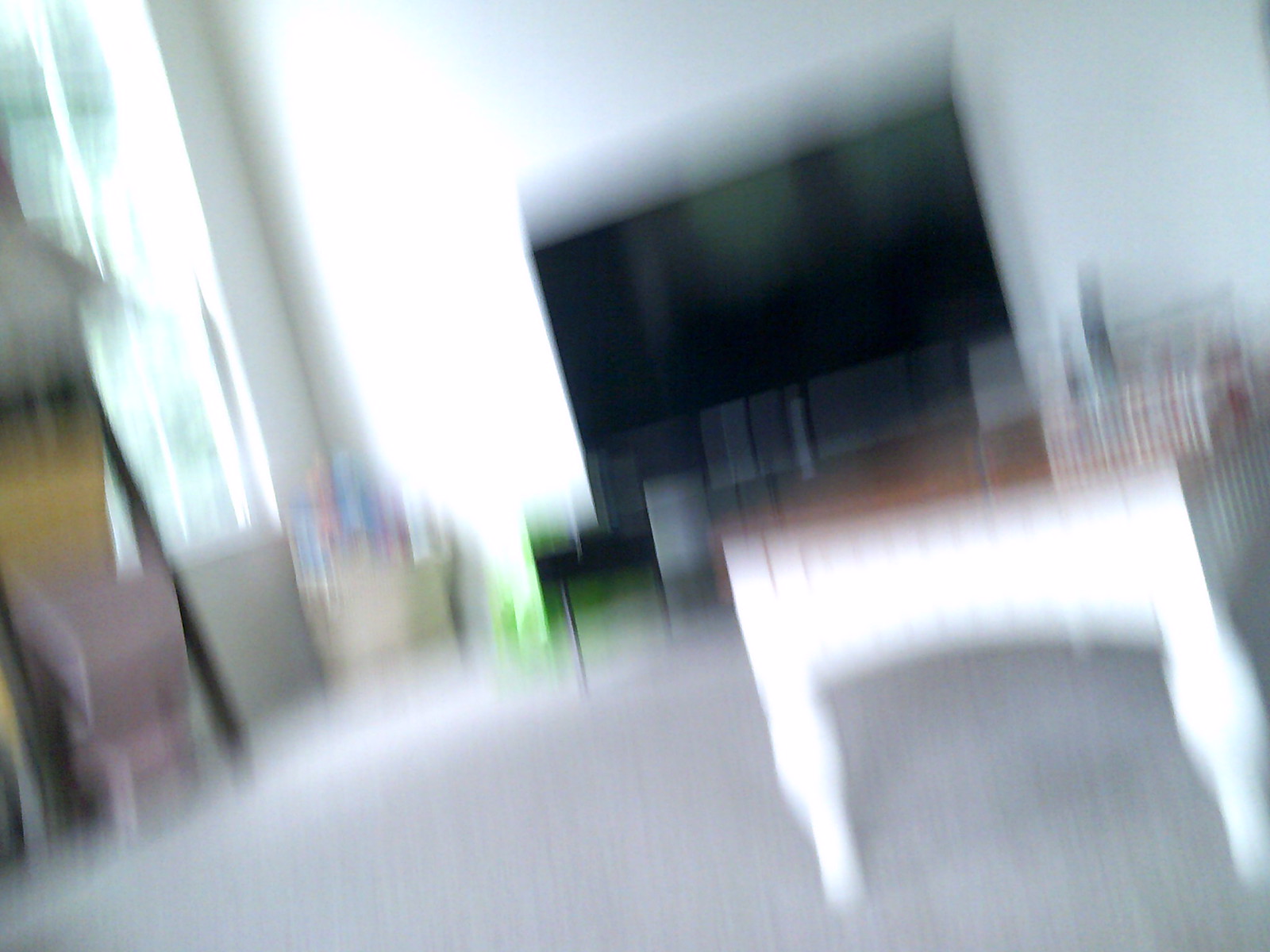A blurry indoor daytime photograph capturing a room in a house with poor focus. Prominently in the background is a large flat screen TV. On the right side towards the foreground, there is a table with white legs and a wooden top, which holds indistinguishable objects. On the left side, a large vertical window allows some light in, though its view is marred by green smudges. Adjacent to the window, on the right, a basket, possibly tan, appears filled with various items. The floor seems to be a light gray color, though the blurriness impacts clarity.